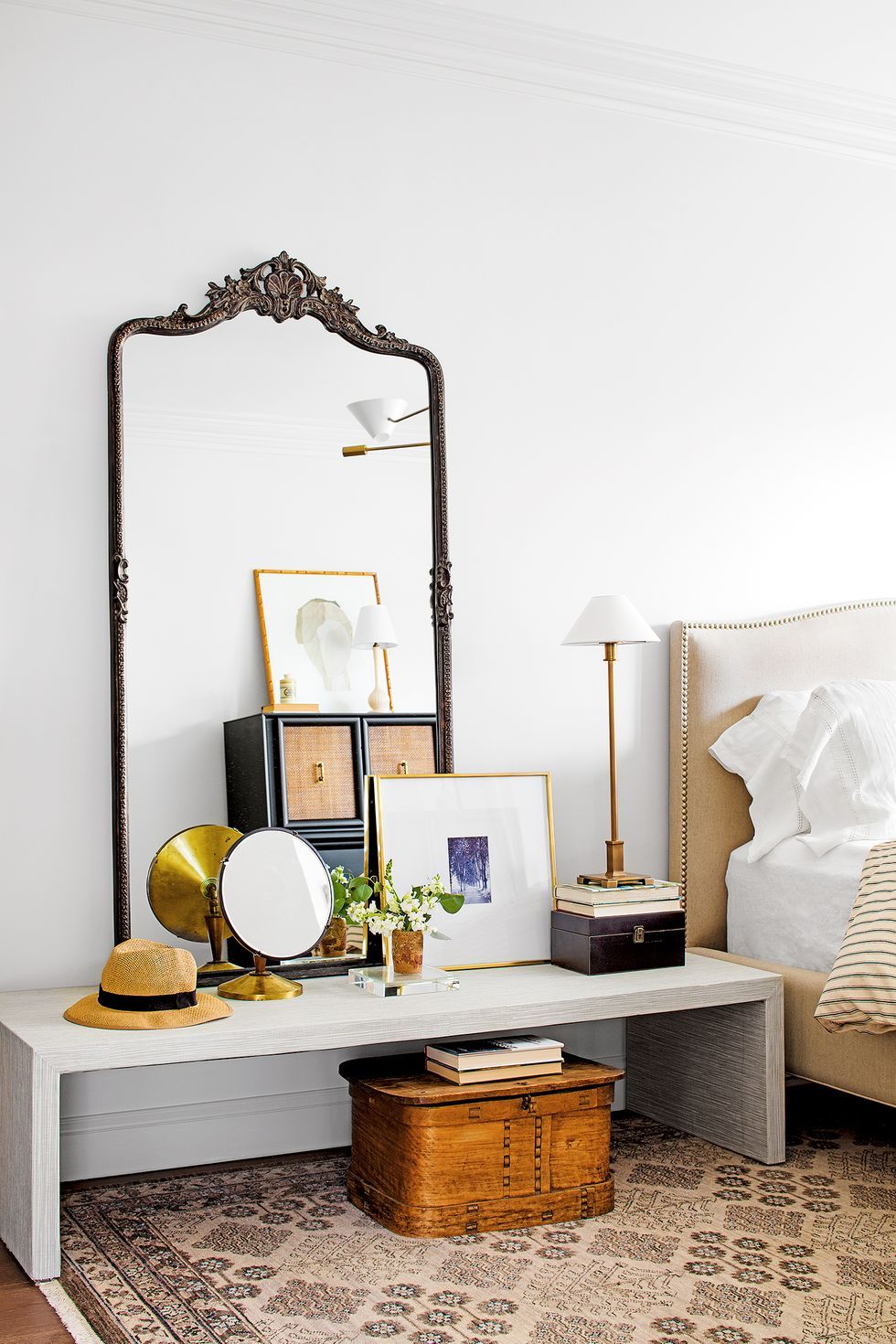This is a detailed photograph of a bedroom with white walls. Dominating the room is a large antique mirror, painted in a darker color and leaned against the wall, reflecting the furniture in the room. A carpet with tan and brown tones covers the floor. In the reflection, there is a gray bedside table next to the bed, adorned with an array of items: a hat, a magnifying mirror, a tall brass lamp with a white lampshade, a framed art piece, a four-compartment storage drawer, a small trinket box, and a vase with white flowers. Beneath the table sits a wooden basket with two books stacked on top. The bed itself has a prominent headboard with beading details and is dressed with white sheets and a striped tan comforter, showcasing a cozy and stylish interior.